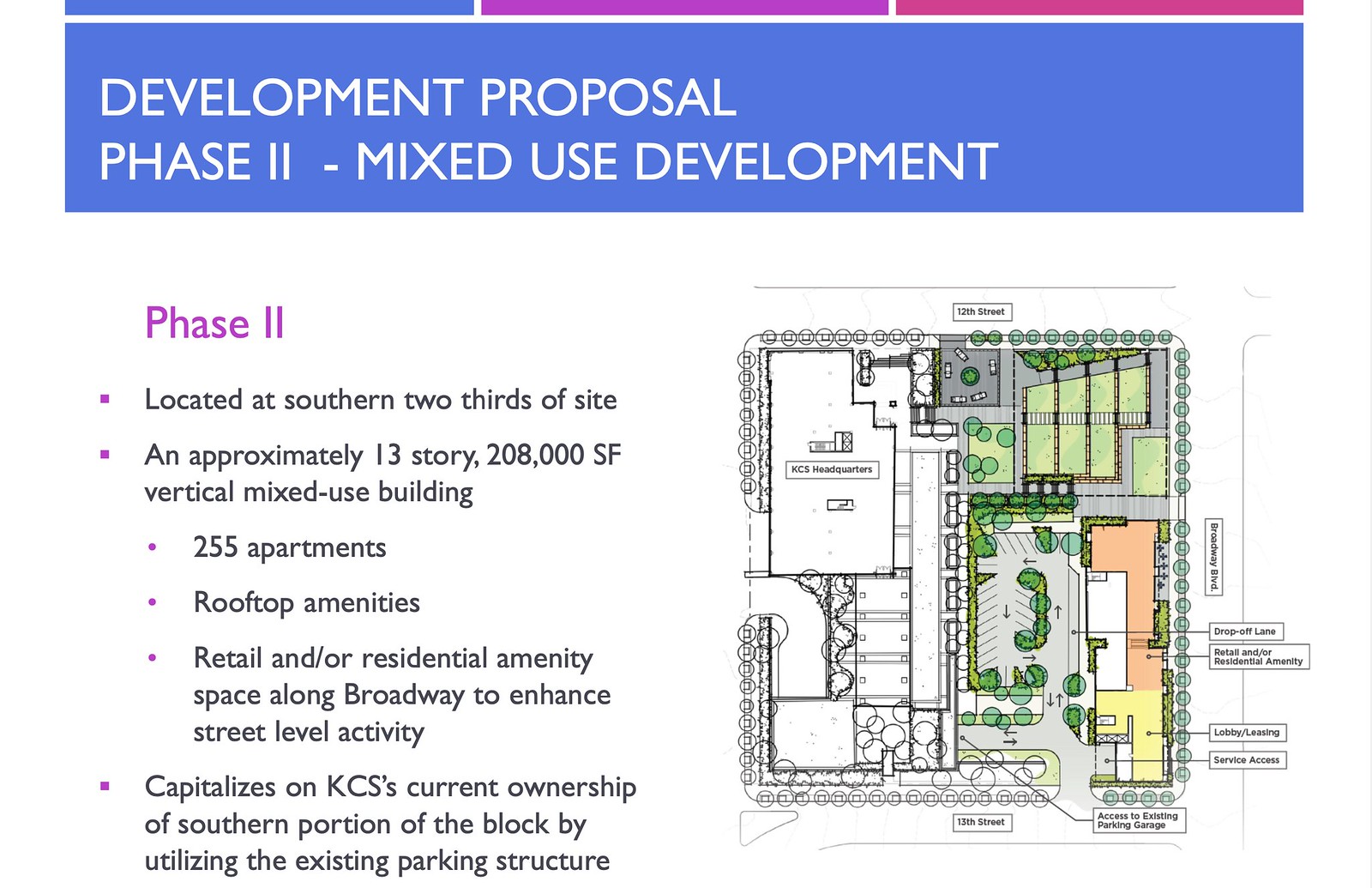The image is a wide rectangular slide from a PowerPoint presentation with a white background. At the top, there is a large blue rectangle containing the title "DEVELOPMENT PROPOSAL PHASE 2 - MIXED USE DEVELOPMENT" in all capital letters with white font. Above this blue bar, there are three thin rectangles in blue, pink, and purple. Beneath the title, the word "Phase 2" is prominently displayed in purple letters. Below this, a detailed bulleted list describes the project: "Located at the southern two-thirds of the site, an approximately 13-story, 208,000-square-foot vertical mixed-use building featuring 255 apartments, rooftop amenities, and retail or residential amenity space along Broadway to enhance street-level activity." It further mentions that the development "capitalizes on KCS's current ownership of the southern portion of the block by utilizing the existing parking structure." On the right side of the slide, there is a comprehensive architectural diagram depicting the building's layout with various colored areas, including green, orange, and yellow shapes, providing a visual plan of the new development.